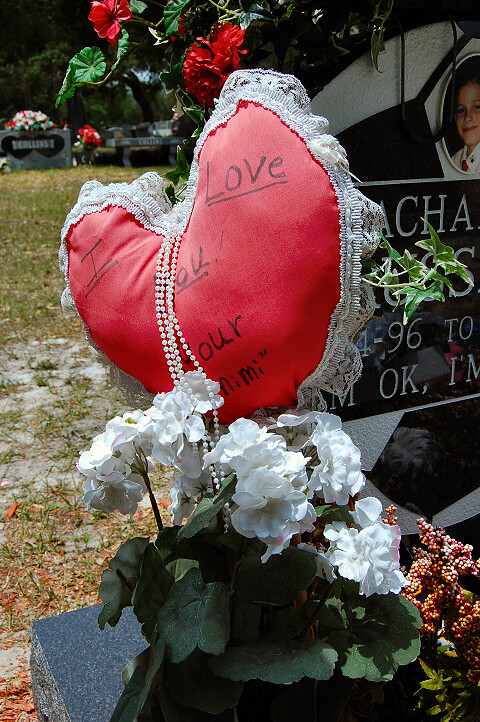This image depicts a serene cemetery scene with green grass as the backdrop. The central focus is a partly visible grey marble headstone on the right side, adorned with various mementos. At the top of the headstone, a child’s portrait is prominently displayed, suggesting a young soul is memorialized here. The text on the headstone that can be discerned includes letters "CHA" and fragments like "A-E-C-H-A-R-U-S-S," "one ninety-six two," and "M-O-K-I-M."

Attached to the left side of the headstone is a red heart-shaped pillow bordered with white fluffy lace. This heart bears the inscription "I love you, you are Mimi," and has a string of pearls elegantly draped from its center, cascading down towards a bouquet of white flowers with green leaves. Red roses with lush green leaves also hang on the tombstone, adding vibrant color to the setting. Additional smaller flowers are visible on the right side of the arrangement. 

In the background, the tranquil cemetery continues with other headstones and floral tributes, accompanied by sprawling lawns and distant trees, adding to the peaceful atmosphere.